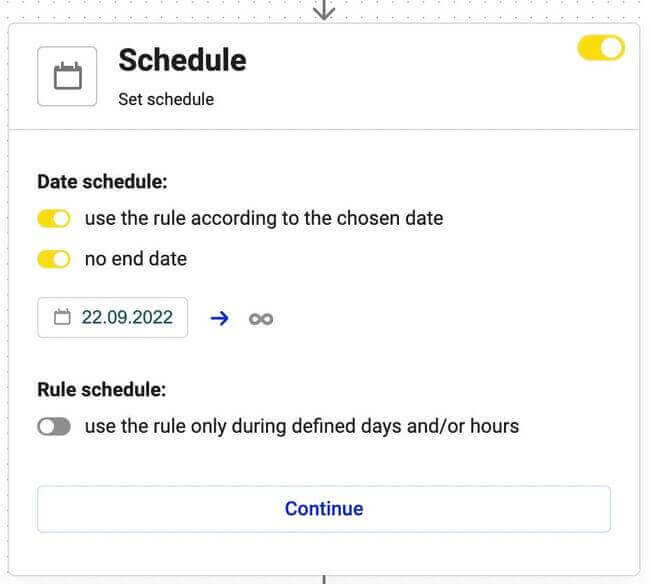This screenshot displays a detailed view of a scheduler pop-up box. In the upper right corner, a toggle switch is positioned and turned on. Directly below it, the word “Schedule” is presented in bold black letters. Beneath this, the phrase “Set Schedule” is accompanied by a calendar icon situated to its left.

Further down, the text “Date Schedule:” is followed by a toggle switch that is also turned on. To the right of this switch, the instruction “Use the rule according to the chosen date” is clearly written. A subsequent toggle switch below is activated, beside the label “No end date.”

Below these switches and descriptive lines, a specific date “09-22-2022” is enclosed within a box. Adjacent to this box, a blue arrow points to the right towards an infinity symbol, symbolizing an ongoing or continuous schedule.

Further below, “Rule Schedule:” is emphasized in black lettering. Alongside this title, another toggle switch is visible but toggled off. Next to this switch, the guideline “Use the rule only during defined days and/or hours” is provided for additional user instructions.

Finally, spanning the entire width at the bottom of this popup box is a prominent and large “Continue” button, encouraging users to proceed with their scheduling settings. This extensive detailing ensures a clear understanding of the various scheduling components and functionalities within the screenshot.